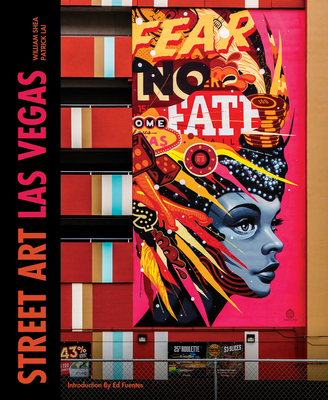The image is a detailed promotional poster for the Street Art Las Vegas festival. It prominently features a vertical black strip along the left side with the label "Street Art Las Vegas" in orange and pink all caps, accompanied by the names of artists William Shea and Patrick Lai in smaller sans serif orange font. At the bottom of the strip, there is an orange sans serif text that reads, "Introduction by Ed Fuentes."

The right side of the poster showcases a vibrant illustration of a woman with a light blue face and a striking, multicolored headdress, which includes feathers, casino chips, the iconic "Welcome to Fabulous Las Vegas" sign, and more eclectic elements. Her headdress is vivid with various colors including pink, yellow, and orange. The text "Fear No Fate" is also integrated into the artwork. The woman is depicted wearing a dark turtleneck, and the background of her portrait is pink.

The poster gives the illusion of being part of an outdoor graffiti mural on the side of a building, with a netted barricade railing visible at the bottom. The lower part of the wall, decorated with vertical stripes in white, blue, brown, and red, features some partially visible food or restaurant posters, including one with "43%". Overall, the poster fuses urban street art with vibrant promotional elements, capturing the essence of Las Vegas’s eclectic culture.